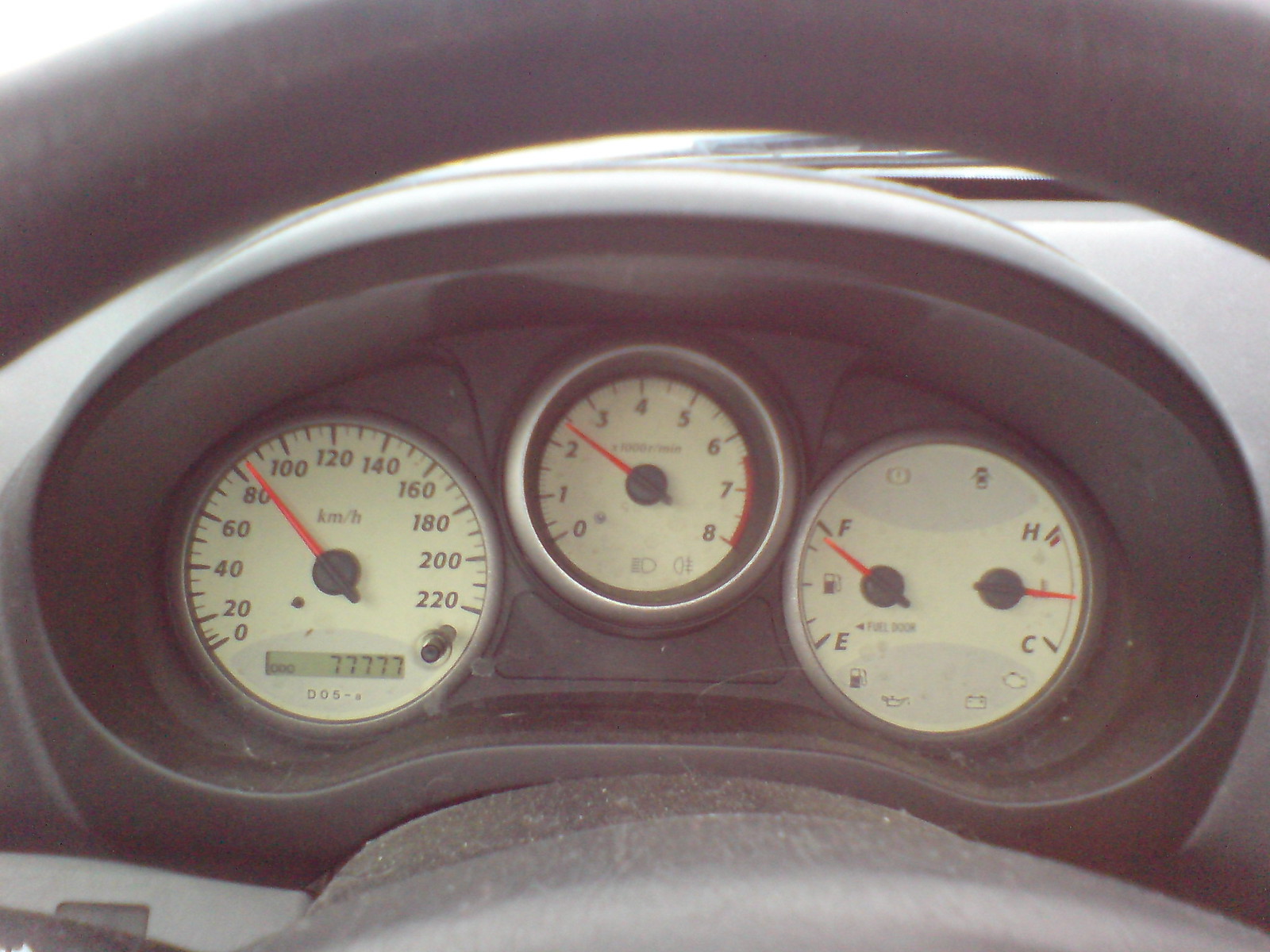The photograph captures a rectangular view of a car's dashboard, predominantly displaying the gauges and the top portion of the steering wheel. The steering wheel, positioned at the bottom center of the image, is visibly coated with dust, hair, and grime, suggesting the car has not been cleaned in some time. Behind the steering wheel shaft, a glossy black-framed, bean-shaped indent houses three circular gauges.

The gauge on the left features a thin orange needle pointing to 80, surrounded by multiple black numbers and notches. Below this, an LED screen displays the numbers "77777," indicating the car’s mileage or another numerical metric.

The central gauge, smaller than the outer two, also contains multiple black numbers and notches, though specific details are less discernible.

The gauge on the far right is a dual-purpose instrument: one section marked with "H" and "C" indicating temperature levels, likely for the engine, and another section labeled with "F" and "E" along with intermediate notches, representing the fuel level. The detailed composition and state of the dashboard highlight both functional and neglected aspects of the vehicle.